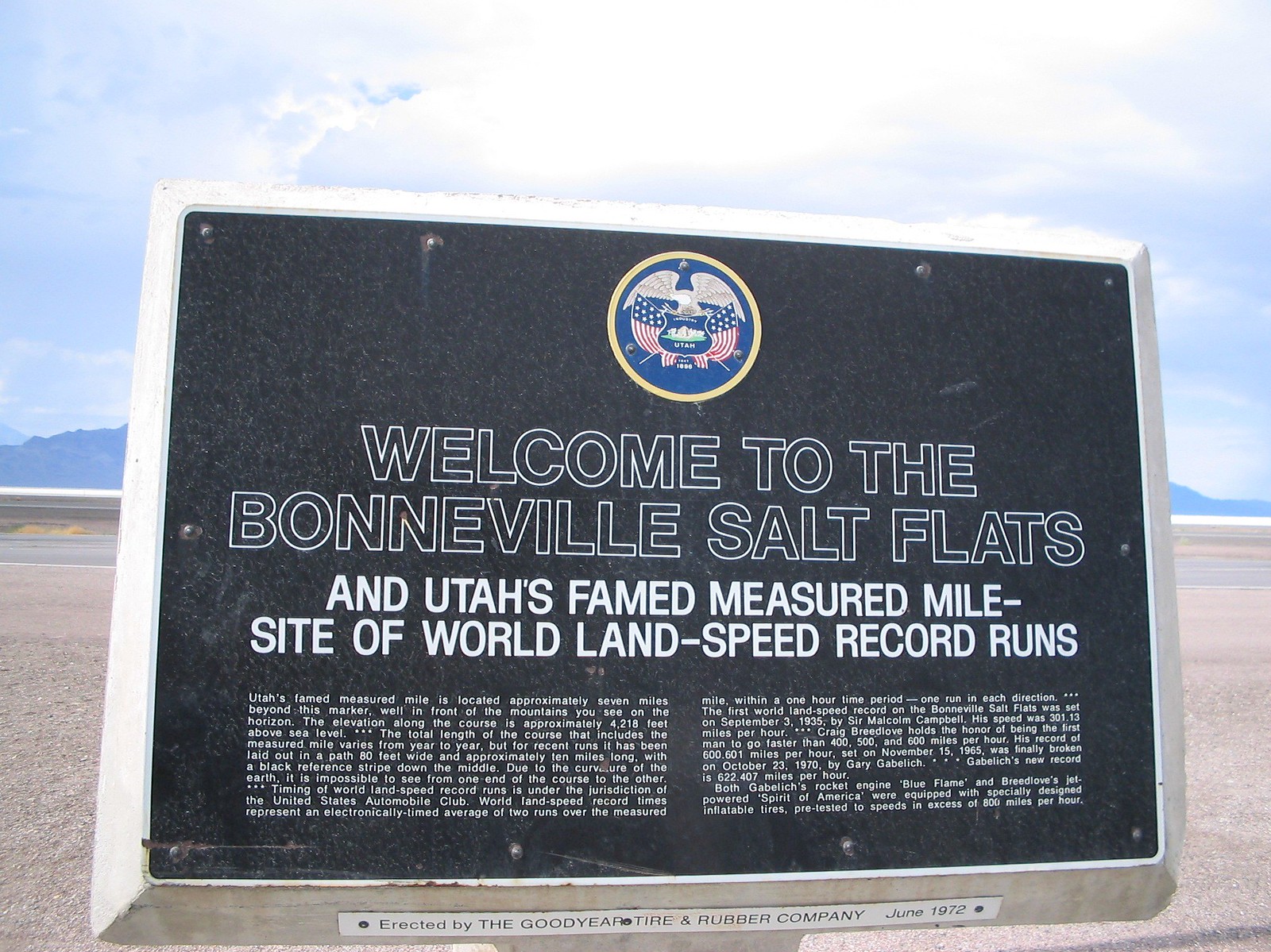The image captures an outdoor scene featuring a worn placard with a detailed introduction to the Bonneville Salt Flats in Utah. Positioned against a backdrop of hazy blue mountains, bright white clouds, and a wide expanse of gray, flat salt ground, the placard is framed by a gray, weathered border. At the top, it prominently displays the seal of Utah, adorned in red, white, blue, and gold colors. The text on the placard reads, "Welcome to the Bonneville Salt Flats" in black with a thin white border, followed by "Utah's famed measured mile site of world land speed record runs." Below this, there is a smaller, hard-to-read text block providing historical information. Additionally, a silver plaque is mounted at the bottom with three bolts, inscribed, "Erected by the Goodyear Tire and Rubber Company, June 1972." The scene is lit by a bright, sunny day, enhancing the clarity and visibility of the surroundings and the placard's details.